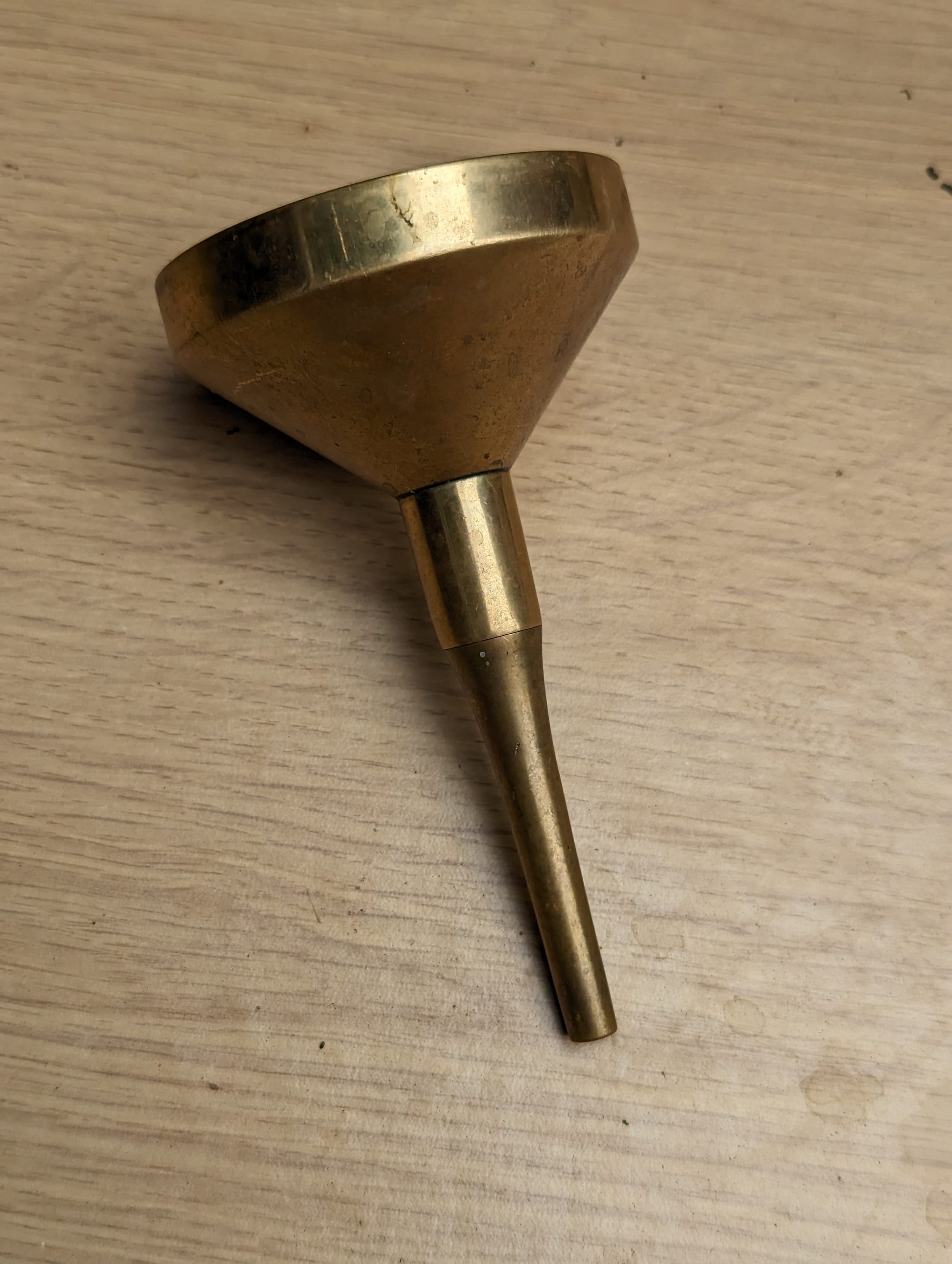This photo captures a small brass object, primarily resembling a vintage perfume funnel, resting at a diagonal angle on a worn wooden table. The funnel, showing signs of age and use, has a bowl-shaped top that narrows into a long, slender stem, much like an old-fashioned metal golf tee. The background consists of an aged wooden surface, marked with years of use, which accentuates the antique appearance of the brass funnel positioned to display its underside rather than through its opening. The grain and lines of the brown wood surface enhance the nostalgic and rustic feel of the scene.